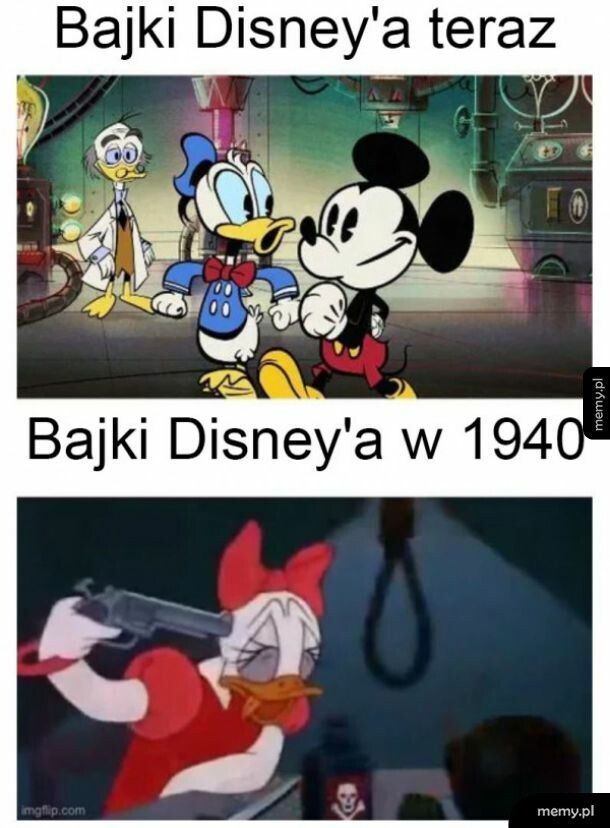A stacked image with two distinct cartoon scenes featuring Disney characters is shown. The top image displays Donald Duck and Mickey Mouse in the foreground, situated in a laboratory setting characterized by scientific equipment including stoves, a large pipe, and a pink lamp post. Donald sports his usual blue hat, red bow tie, blue shirt, and has his yellow beak prominently visible, while Mickey is seen with his red pants, yellow shoes, white gloves, and signature black ears and smile. Behind them, another character, resembling Uncle Scrooge, is dressed in a white lab coat with gray hair at the sides, working amidst this detailed, lively lab environment. The text above this scene reads, "Boschki, B-A-J-K-I, Disney, a teraz, T-E-R-A-Z."

The bottom image features Daisy Duck, distinguishable by her pink bow and red-pink dress, in a dramatically darker setting. She appears to be in distress, with a gun pointed to her head and a menacing noose hanging from the ceiling beside her. In front of her lies a table with ominous objects including a poison bottle marked with a skull and crossbones. The caption below this tense scene says, "Boschki, B-A-J-K-I, Disney, W 1940." The overall composition combines classic Disney animation with surprisingly macabre elements, captured in a vividly detailed cartoon style.